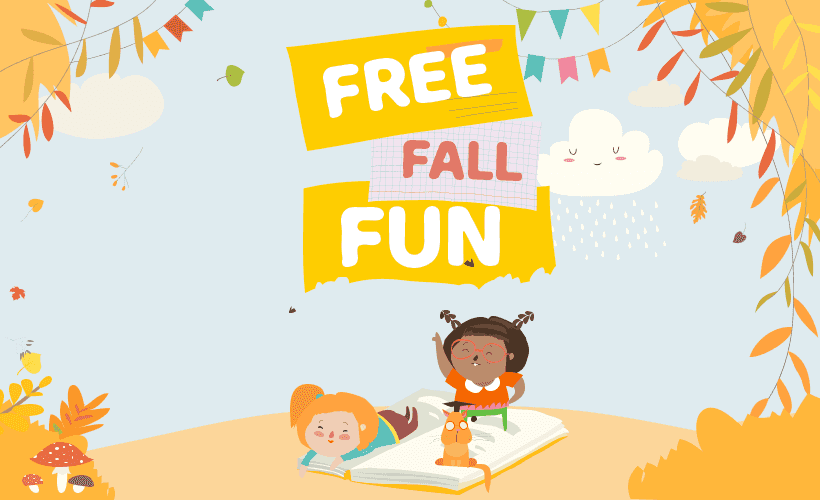This image shows a colorful, cartoon-style advertisement for a fall event. Dominating the illustration are vibrant yellow and red leaves that frame the scene, indicating an autumn setting. The central text, written over yellow brush strokes, reads "Free Fall Fun." The sky in the background features light blue hues with whimsical clouds, one of which has closed eyes and appears to be gently raining, though no one seems to be getting wet.

On the ground, the scene centers around two young girls on a large book. One girl, who seems to be African American with brunette hair, is sitting up and holding something green. The other girl, who has blonde hair, is sitting down wearing a blue shirt and red pants. Near them, a quirky squirrel is perched at the edge of the book, mouth open, perhaps chattering in delight. Adding to the cozy fall atmosphere, the bottom left corner of the image shows a cluster of mushrooms—two orange and one red—growing amidst the scattered leaves.

The overall composition, rich in details like leaves, sky, and clouds, invites viewers to a whimsical, fall-themed event filled with fun and nature.